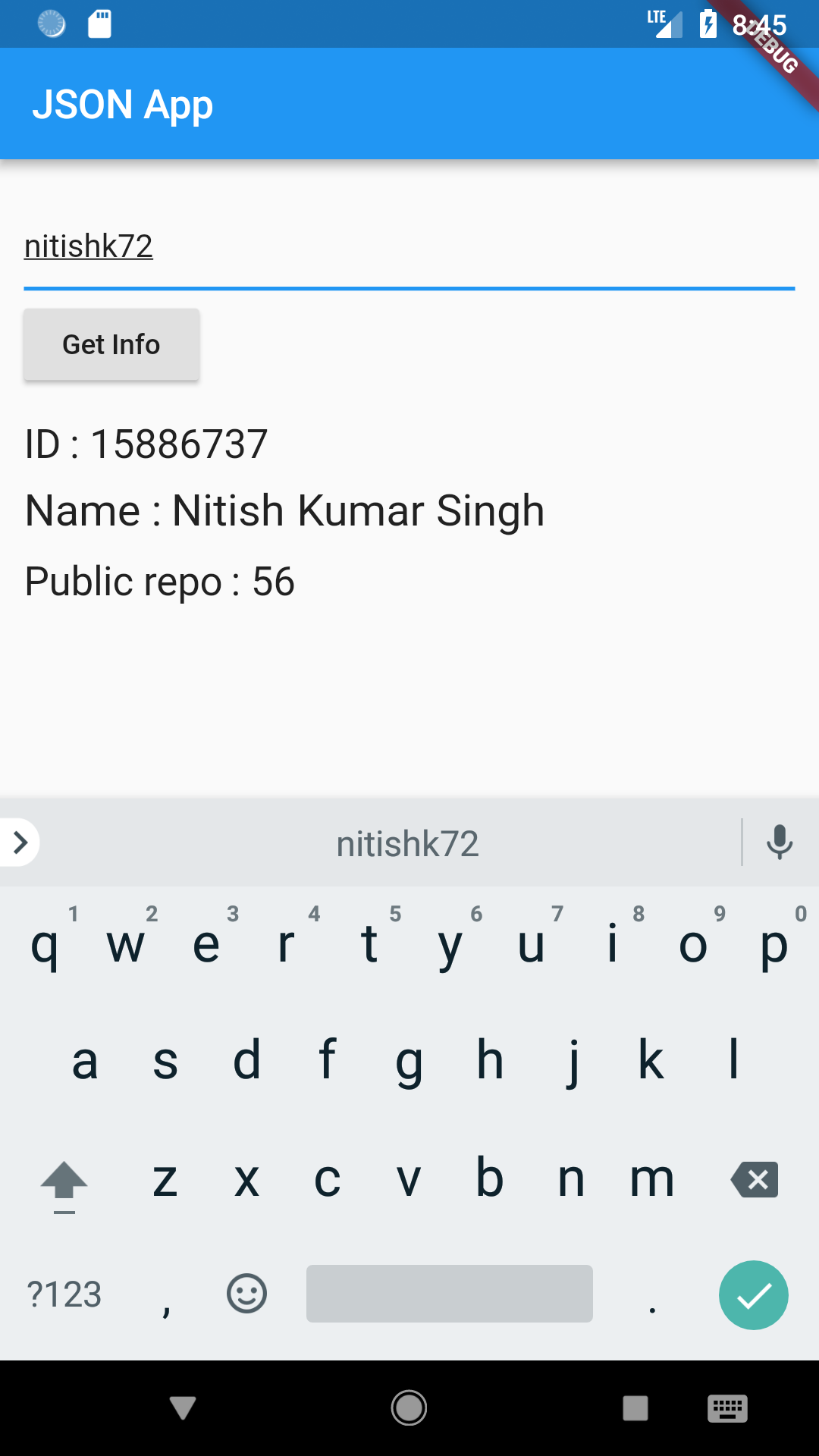A smartphone screenshot displays detailed application information at 8:45. The phone has either two or four signal bars, and the screen features a light blue border at the bottom labeled "JSON app." Above this border, the screen has a white background with a blue horizontal line bearing the username "NITISHK72." Below this, a gray rectangle prominently displays the button labeled "Get Info." Further details include "ID: 15886737," "Name: NITISHKUMAR SINGH," and "Public Repo: 56," sequentially listed. A text box containing "NITISHK72" and a microphone icon on its right is situated just above the on-screen keyboard. The bottom of the screen features a black bar with three icons: a triangle (probably a 'back' button), a circle (home button), and a gray square (recent apps).